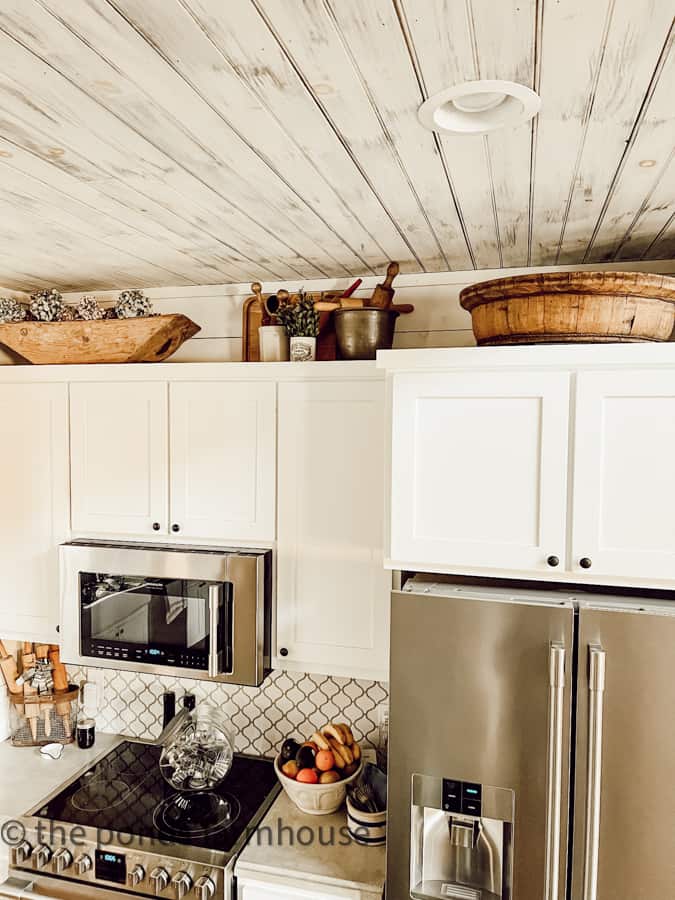This detailed aerial view of a kitchen showcases a variety of elements, from appliances to cabinetry. In the bottom left corner, text along with a copyright symbol appears, albeit blurry and difficult to read. The kitchen layout includes a black-surfaced induction stovetop with a stainless steel front, which is flanked by a marble-like countertop. Above the stovetop, a silver microwave is seamlessly integrated into the wall cabinets. These cabinets are white with black knobs and are adorned with wooden baskets, a small potted plant, and kitchen utensils such as rolling pins on top. Just to the right of the stove is a bowl of fruit. The kitchen also features a double-door stainless steel refrigerator, complete with an ice and water dispenser on the left door. The countertop's backsplash displays a black and white lattice pattern, adding a touch of elegance to the room. The ceiling above appears to be made of painted white floorboards.